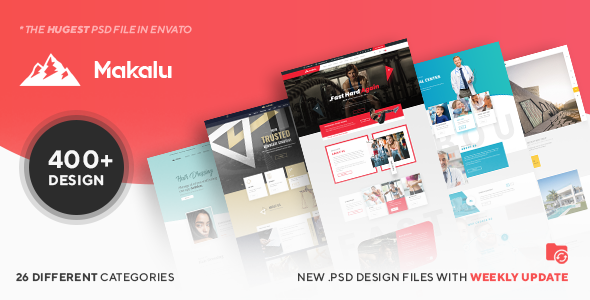**Makalu Design Advertisement**

Introducing Makalu, the ultimate resource for designers and creators, proudly showcased in pristine white text against a dynamic, swooping red background. At the heart of the visual is the Makalu logo, a sleek white graphic of a mountain, representing the pinnacle of design excellence. Right above the logo, the bold claim "The Hugest PSD File in Envato" captures your attention immediately.

Centered below the logo, a striking black circle highlights a remarkable feature: "400+ Designs." This eye-catching element is complemented further by the text at the very bottom. On the left, in black text, it emphasizes "26 Different Categories." Adjacent to it, more black text announces "New .PSD Design Files," punctuated by red text that proclaims "Weekly Update." An intuitive file icon with a reload symbol reinforces the idea of consistent, fresh updates.

Just above this section, your eyes are naturally drawn to a vivid display of five small images. They resemble magazine or website layouts, arranged in an engaging, overlapping fashion. The central image is placed slightly higher with two images flanking it, their edges partially concealed, creating a cascading visual effect. Beneath this trio, two more images sit, similarly overlapped, as if floating gracefully above one another. These images showcase a variety of designs in vibrant red, blue, and white hues, hinting at the diverse creative possibilities within Makalu.

Discover the boundless potential of Makalu, where creativity meets cutting-edge design!